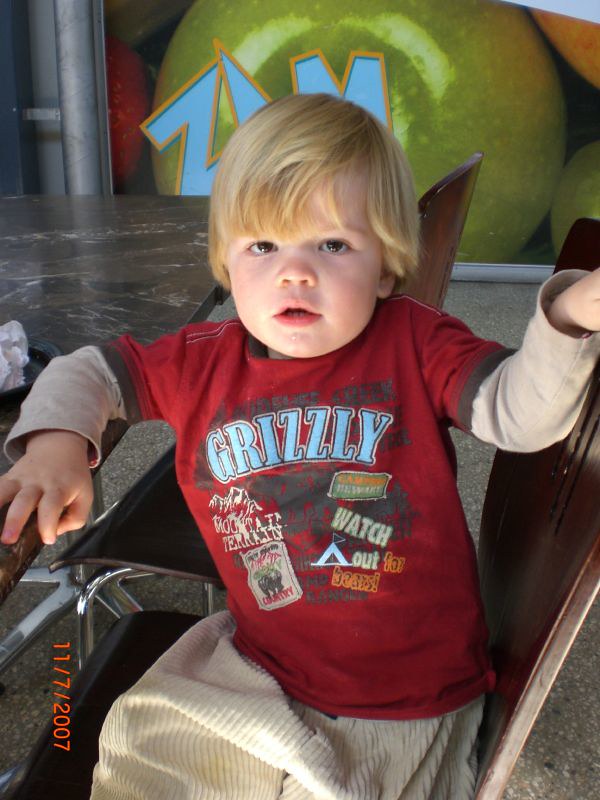This is an image of a young blonde boy, likely a toddler, seated at an outdoor stone table. The table is grey, and he’s using it for support. The boy wears a red t-shirt over a white thermal shirt, with the text "Grizzly" emblazoned in white across his chest. He appears to be sitting on a brown wooden chair and has a beige blanket draped over his lap. His haircut resembles that of Boris Becker, and he is looking directly at the camera. Behind him, there is a large advertisement featuring a big green apple, suggesting the setting could be a fair or another public event rather than his home. There is no one else present in the photograph. The image is slightly taller than it is wide, and in the lower-left corner, the date "11-7-2007" is visible, indicating when the photograph was taken.